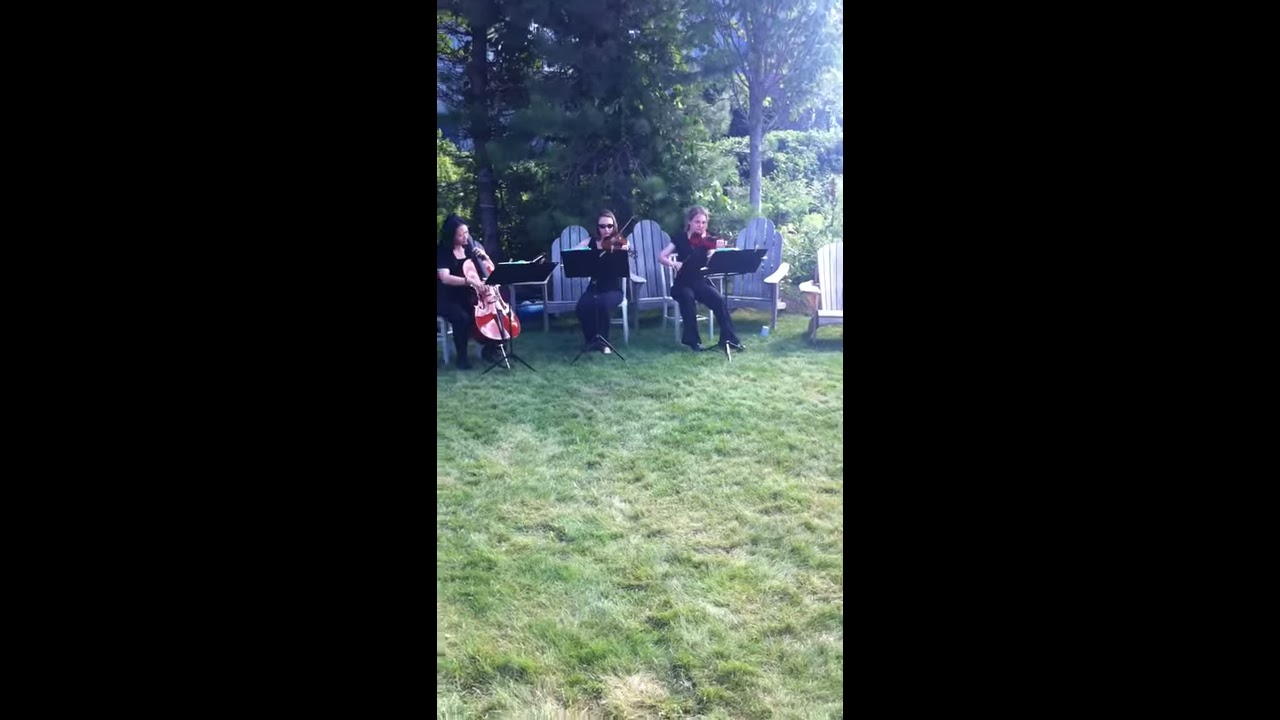The image is divided into three panels, with the outer panels being entirely black and the central panel capturing a detailed outdoor scene. The centerpiece photograph features three musicians seated on a grassy lawn in a backyard setting. Each musician is engrossed in playing a stringed instrument, with the woman on the left playing a cello. She is dressed in a short-sleeved black shirt and black pants. Next to her, in the center, is a blonde woman with either sunglasses or glasses, dressed in black jeans. Though her top is obscured by a music stand, she appears to be playing a violin. The rightmost musician also seems to be playing a violin and is another blonde woman, similarly dressed in a short-sleeved black shirt and black pants. All musicians have music stands holding sheet music in front of them, partly obscuring their upper bodies.

The foreground is a patchy lawn, with vibrant green grass interspersed with dried patches. Behind the musicians, there are several white lawn chairs with high backs, blending into the scene. Further back, the yard is framed by tall trees and bushes, contributing to the serene and somewhat sunny atmosphere, though the sky itself is not visible.